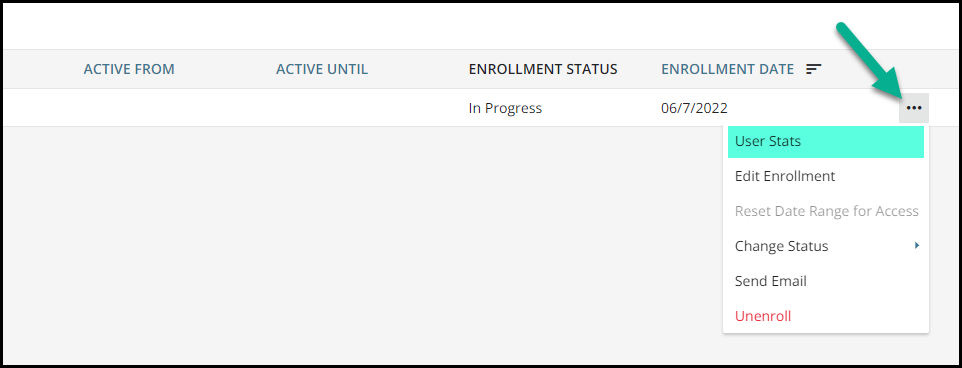This image is a screenshot of a software interface, likely part of a tutorial. The design features a horizontal rectangle with a black outline. The background is primarily gray with white sections. On the right side, there are three black dots arranged vertically, which seem to be a focal point emphasized by a green arrow pointing at them.

On the left side, there's a green bar labeled "User stats," highlighted to draw attention. Below this bar, a dropdown menu has been activated, listing several options:
- User stats (highlighted in green)
- Edit enrollment
- Reset date range for access
- Change status
- Send email
- Unenroll (in red)
- Active from (with no date specified)
- Active until (with no date specified)
- Enrollment status: In progress
- Enrollment date: 6-7-2022

The purpose of the green arrow and the green highlighting suggests this image is a step in a tutorial, guiding the user on how to access user stats.

The color palette includes various shades: blue, white, gray, green, turquoise, black, and red.

Overall, this image appears to instruct users on navigating and managing user statistics within the software.